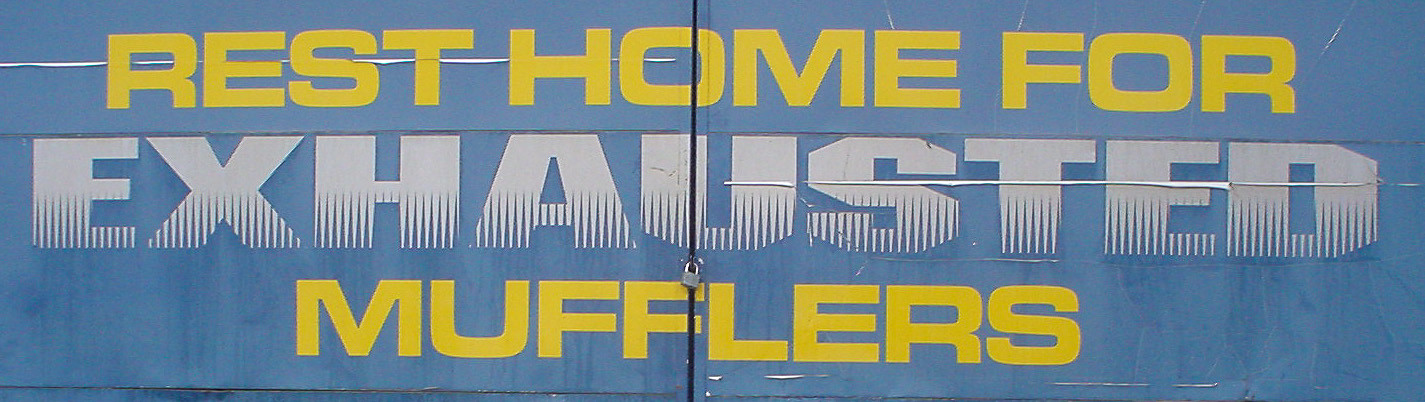This image showcases a rectangular sign predominantly featuring the colors blue, white, and yellow, likely situated on the back of a truck or a doorway, potentially acting as a banner or bumper sticker. The background is light to medium blue, accentuated by faded dark blue stripes that create a running paint effect. At the top of the sign, in bold yellow capital letters, it reads "REST HOME 4." Below that, in even larger, spaced-out white capital letters, it displays "EXHAUSTED," with subtle blue lines extending from the bottom of each letter. At the bottom, again in yellow capital letters, it says "MUFFLERS." Notably, there is very minimal spacing between the words "REST HOME 4" and "MUFFLERS." The image also features details like a horizontal white line, some pilling in the lettering, and the presence of a padlock, reinforcing the sign's attachment, possibly indicating its installation on a mechanical door or vehicular surface. The overall impression is that of a detailed and visually textured advertisement, with REST HOME 4, EXHAUSTED, and MUFFLERS prominently highlighted in their respective colors and sizes.